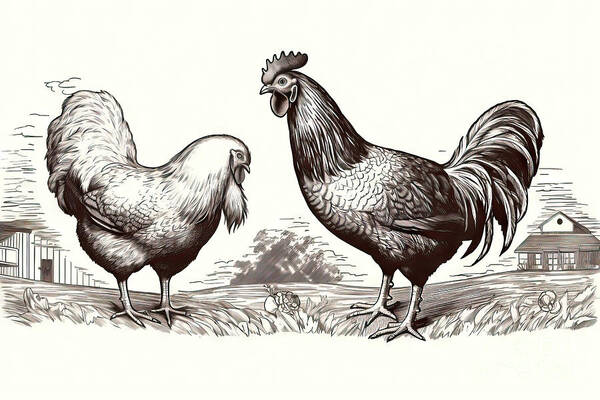This detailed black and white, horizontally rectangular drawing depicts a serene farm scene without definitive borders or background. Dominating the foreground are a large, healthy rooster and a slightly smaller hen, both meticulously rendered with abundant plumage. The rooster, standing on the right and facing left, has its head upright with distinctive flaps above and below its beak, while the hen, on the left, gazes downward. Between them lies what appears to be a broken egg, capturing their attentive stances.

Behind the poultry scene, one can discern more of the farm setting. The lower right corner reveals a farmhouse with a second story and a prominent round window peeking out. On the lower left side of the image is a partial view of another building, possibly a barn, with vertical lines and windows, although its full structure remains indistinct. The ground appears grassy.

The atmosphere hints at a vintage or earlier decade, with touches of sepia in the sky suggesting subtle clouds to the far left, contrasting the otherwise black, gray, and white tones of the scene. This detailed sketch emphasizes a tranquil moment on a farm, centered around the sharply-drawn rooster and hen amidst their simple, rustic surroundings.